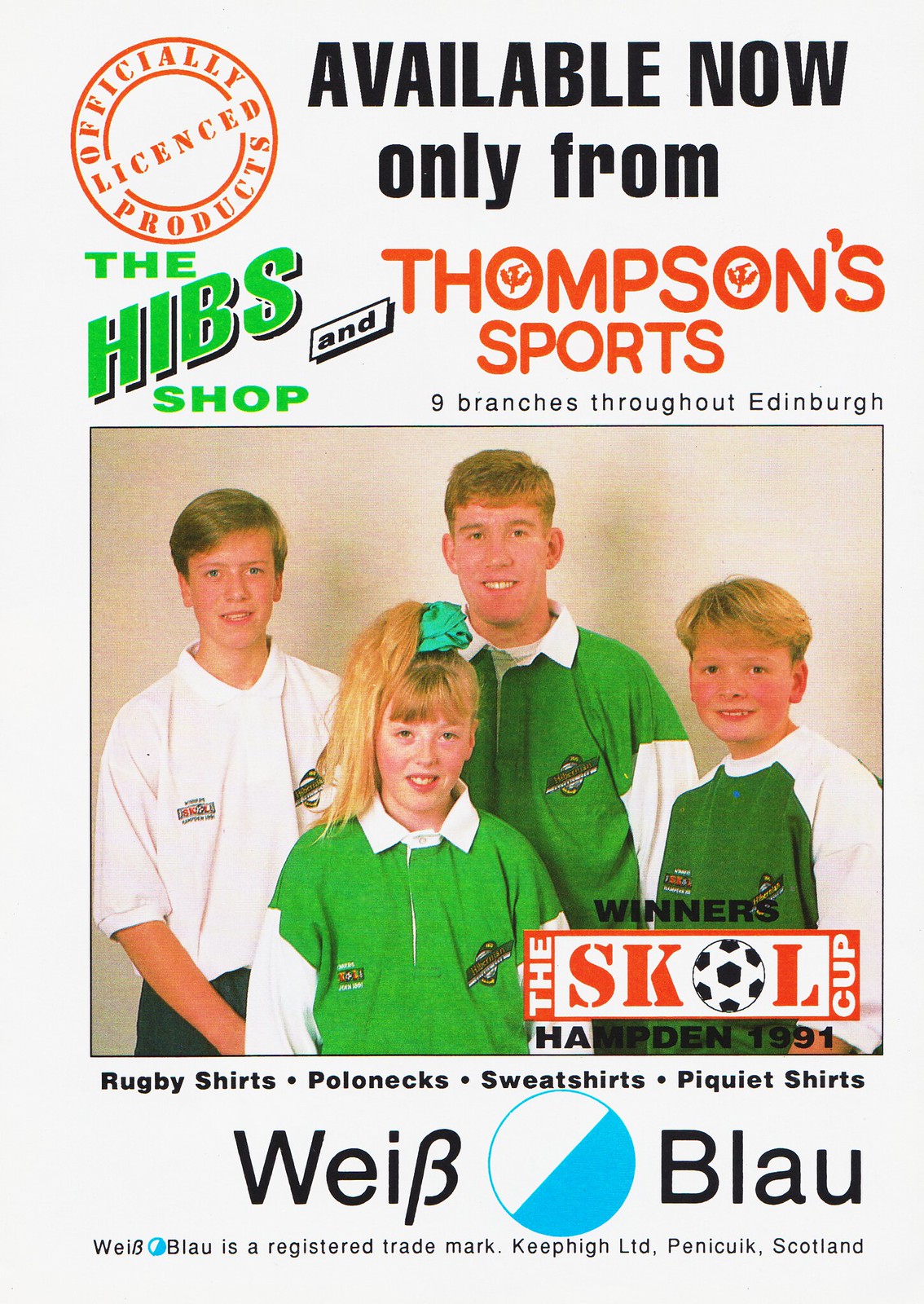The image is an advertisement for the Hibbs Shop, officially known as H-I-B-S, specializing in sports apparel. The ad appears on a magazine page. It prominently features four youngsters—three boys and one girl—all dressed in athletic gear. The girl and two boys are wearing green rugby shirts with traditional white collars, while the boy on the left is in a white polo shirt, and the boy on the right is in a pullover. Above the picture are the words "Officially licensed products," encased in a red-orange circle. The text states that these items are exclusively available from Thompson's Sports and the Hibbs Shop, which have nine branches throughout Edinburgh. Notable items listed in bold text include rugby shirts, polo necks, sweatshirts, and piquet shirts. Overlaying the image is a logo noting "Hampton 1991, the Skull Cup winner," suggesting a vintage 90s style. Near the bottom, the term "Weeb Blau" (W-E-I-B-B-L-A-U) appears, marked as a registered trademark under Kep High Limited, Penicuic, Scotland.